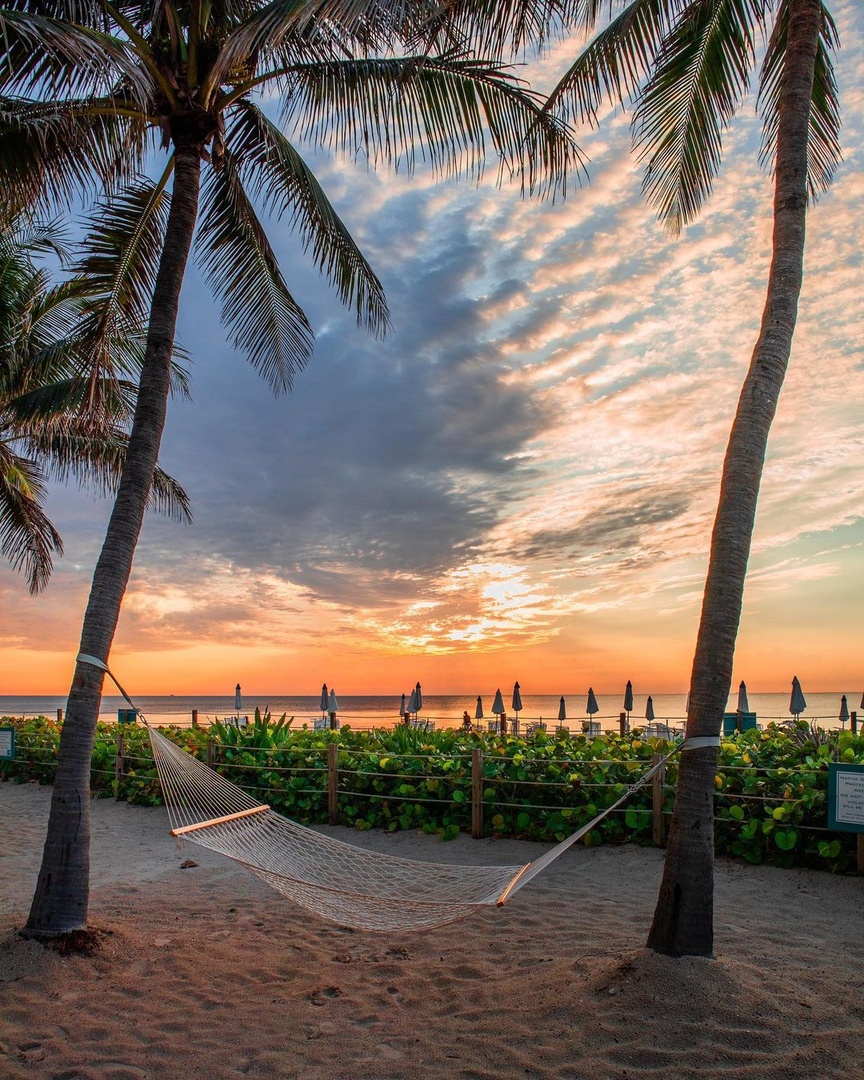The image captures a serene beach scene at sunset, anchored by a prominent white mesh hammock adorned with golden designs at the top and bottom. This hammock is gracefully suspended between two green palm trees emerging from sandy soil, with visible footprints marking the sand. Directly behind the hammock and trees stands a low wooden fence, beyond which lies a garden area with low green shrubs and a dozen or so folded beach umbrellas in darker colors. The backdrop features a tranquil body of water, reflecting the warm hues of the setting sun. The sky transitions from a vivid orange to soothing blue, interspersed with clouds, creating a picturesque blend of sunset colors.